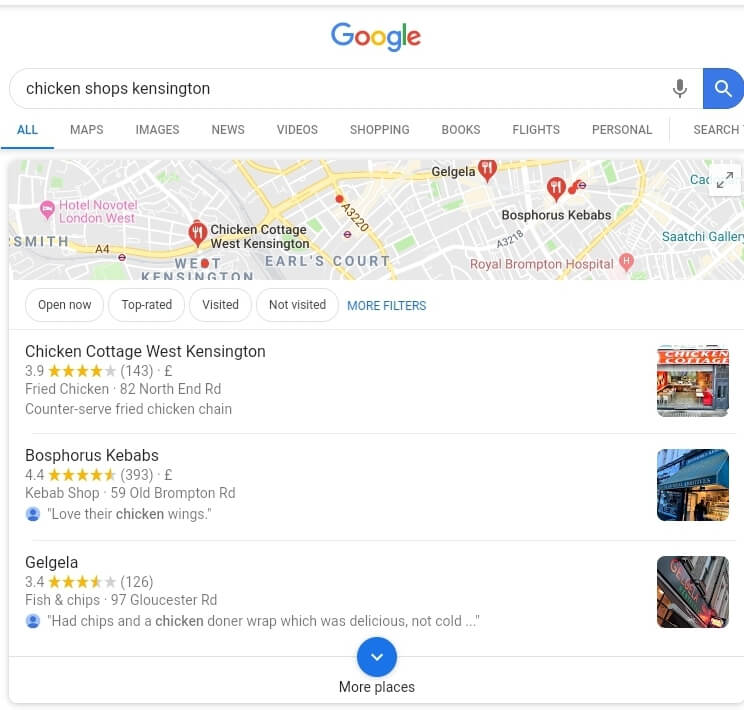The image is a screenshot of a Google search results page that appears on a computer screen. At the top center of the page, the colorful Google logo is prominently displayed above a search bar. The search query entered is "chicken shops Kensington."

Beneath the search bar, a horizontal map spans the width of the page, pinpointing various locations in Kensington, England. The top navigation bar shows the user has clicked on the "All" tab. Listed below the map, several search results are displayed with details of local establishments.

The first result is for "Chicken Cottage West Kensington," which has a rating of 3.9 stars. It is described as a place that offers fried chicken, along with its address. To the right, a square image shows a picture of Chicken Cottage.

The second result features "Phosphorus Kebabs," boasting a rating of 4.4 stars. It is identified as a kebab shop, and a small square image on the right displays the storefront of Phosphorus Kebabs.

The final result at the bottom lists "Gal Gala," with a rating of 3.4 stars, described as a fish and chips shop. An image to the right shows the exterior of Gal Gala.

At the very bottom center of the page, a blue circle with a down arrow indicates the option to "see more places" by clicking on it to reveal additional restaurant listings.